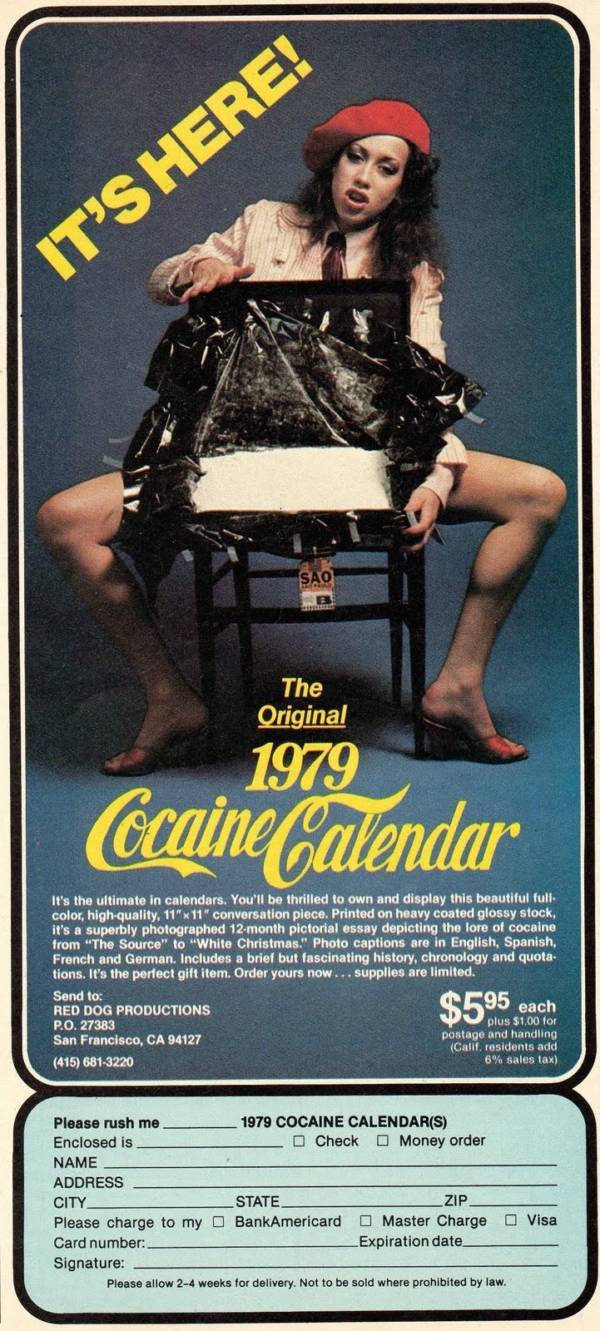The image is a detailed illustration resembling an advertisement, featuring a striking visual of a woman seated on a black chair, facing its back with her legs spread on either side. She is tilting slightly to the left, her mouth slightly open as her long dark hair frames her face. She is wearing a red beret, a light-colored long-sleeve collared shirt, and little red mules. 

In front of her, between her legs, there appears to be a black trash bag and a stark white block. The background of the image is predominantly dark blue, while the top left corner displays the phrase "It's here" in yellow letters. Below the woman, text reads: "The original 1979 cocaine calendar," followed by a paragraph of detailed product information and purchase instructions. There's a blue rectangle at the bottom of the image containing a form with fields to order the calendar, asking to "Please rush me" a certain number of 1979 cocaine calendars, along with spaces to fill in address details.